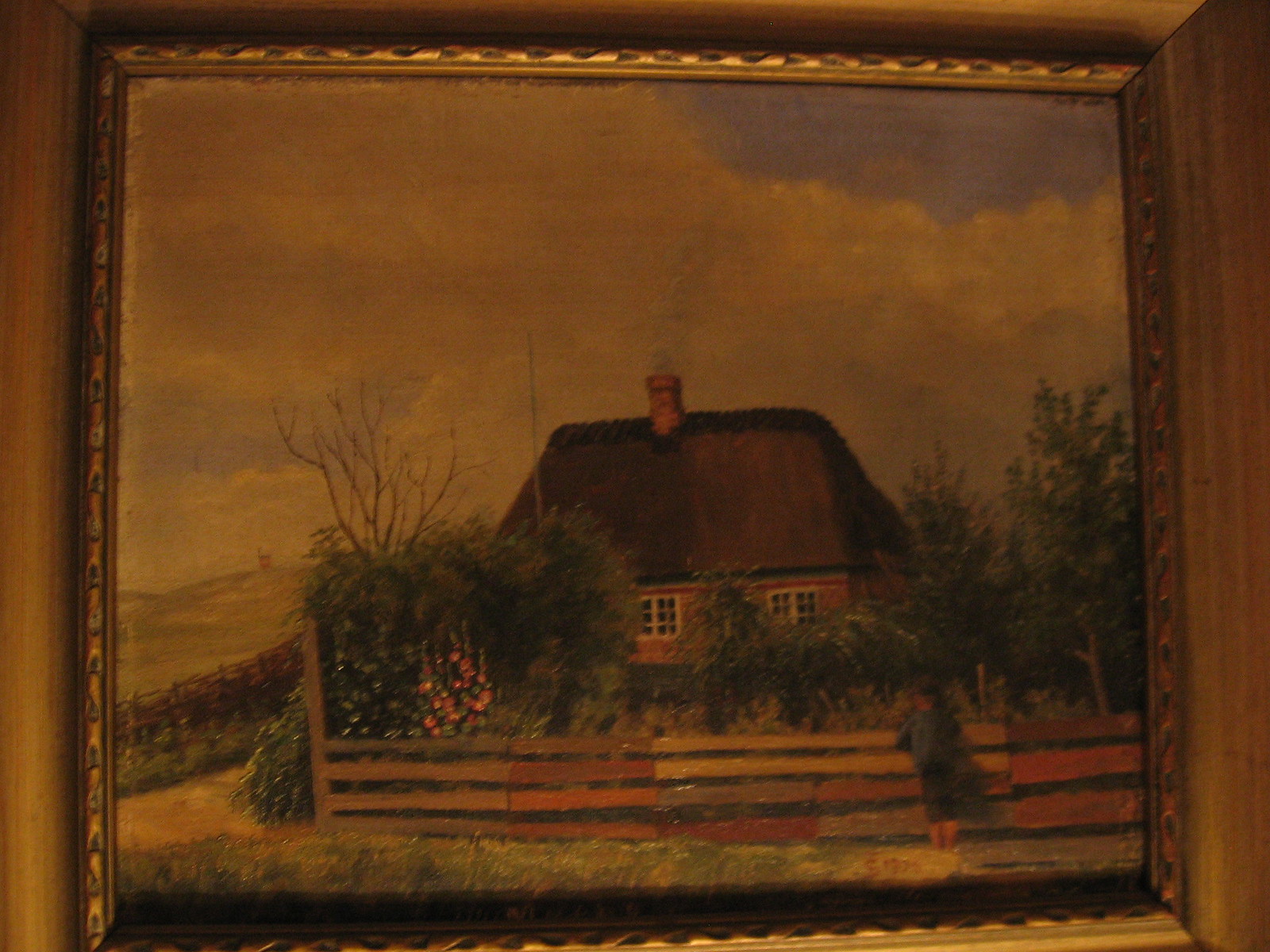The painting, enclosed in a detailed gold-brown wooden frame, captures a melancholic scene predominantly utilizing dark colors. Underneath the frame's warm wooden tones, the dimly lit room adds to the painting's ambience, suggesting it was photographed indoors with a lamp casting warm light from below, hinting at nighttime. The sky in the artwork is heavily clouded and dark, amplifying the overall moody atmosphere.

Central to the painting is a house characterized by its deep red facade, white window frames, and a prominent brown rooftop crowned with a chimney. The house is nestled amidst dark green bushes and lies behind a sturdy wooden fence composed of four horizontal planks fastened together with posts at each end. In the foreground, a young boy stands outside the fence, dressed in a dark navy blue outfit with his back turned, gazing towards the house. Surrounding the scene, the landscape includes a hill on the left and some trees, adding depth to the portrayal of a secluded garden setting.